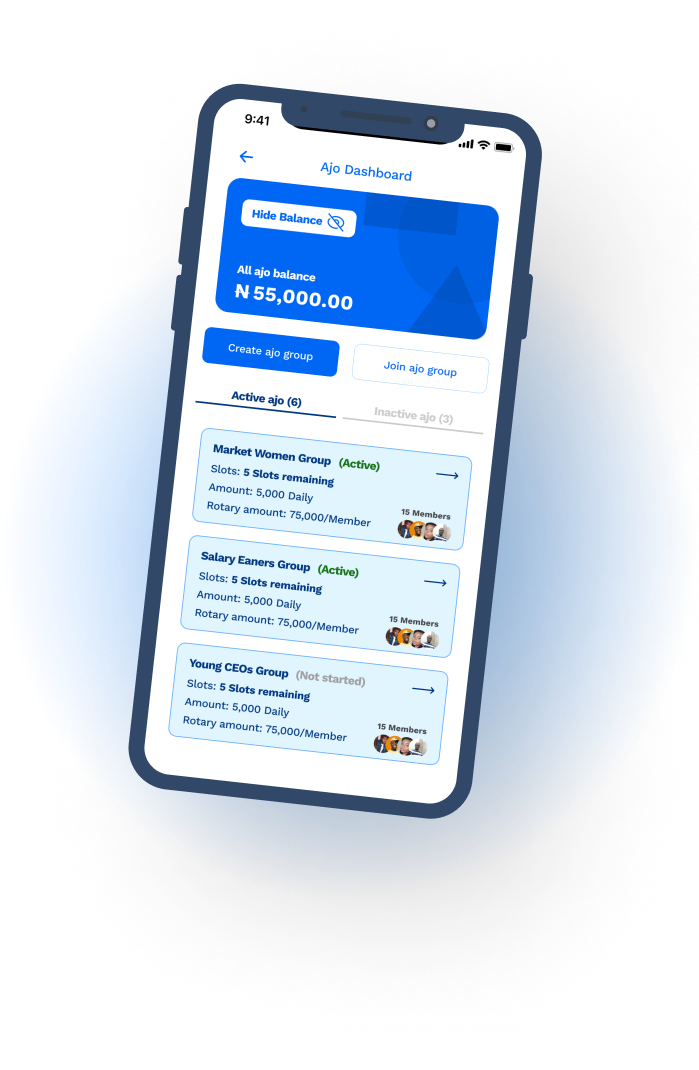The image depicts a smartphone, specifically an iPhone, with a bright white screen backdrop. The top-left corner displays the time "9:41 AM" in black. On the top-right, cellular signal strength shows four bars, Wi-Fi connectivity has three bars, and the battery icon indicates a full charge, all in black.

At the very top, a light blue arrow pointing left is visible, beside the text "Ajo Dashboard." Centered on the screen is a blue card featuring a "Hide Balance" button on the top-left with blue text accompanied by an eye icon crossed out. The bottom left of the card displays "All Ajo Balances" in white, followed by "N55000."

Below the card, two buttons are aligned horizontally. The blue button on the left reads "Create Ajo Group" in white text, while the white button on the right reads "Join Ajo Group" in blue text.

Beneath these buttons, there are two tabs labeled "Active Ajo (6)" in dark blue on the left and "Inactive Ajo (3)" in gray on the right.

Further down, three light blue rectangular bubbles list different groups with their respective details:

1. **Market Woman Group** - Status: Active, Slots Remaining: 6, Amount: 5000 Daily, Rotary Amount: 75,000 per member.
2. **Salary Earners Group** - Status: Active, Slots Remaining: 5, Amount: 5000 Daily, Rotary Amount: 75,000 per member.
3. **Young CEOs Group** - Status: Not Started, Slots Remaining: 5, Amount: 5000 Daily, Rotary Amount: 75,000 per member.